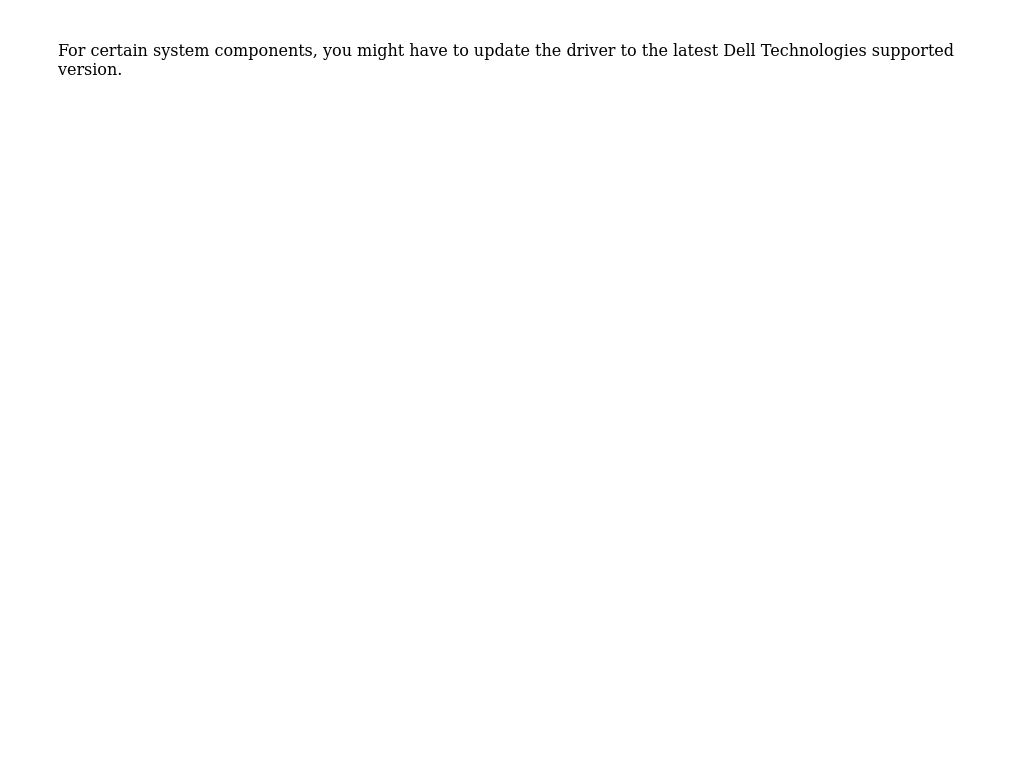The image is predominantly blank, featuring an expansive white background that seamlessly blends with the adjacent white display screen. At its center, a single, succinct sentence stands out in stark contrast to the emptiness surrounding it. The sentence reads: "For certain system components, you might have to update the driver to the latest Dell Technologies supported version." This message, originating from Dell Technologies, suggests a need to update specific system component drivers to maintain compatibility and functionality. The image lacks any interactive elements, such as buttons or links, and provides no additional context or instructions for performing the update, emphasizing the solitary nature of the displayed sentence. This minimalistic presentation highlights the common and often frustrating experience of encountering vague tech support messages that offer limited guidance.